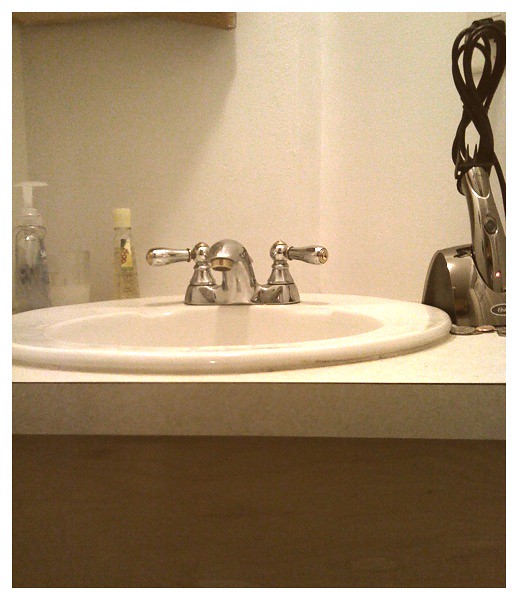The image captures a close-up of a bathroom corner featuring a simple white sink basin. The sink is embedded in an off-white countertop that appears to have wooden cabinets beneath it. Positioned around the sink are four noticeable items, enhancing the otherwise unembellished scene. A clear bottle of Softsoap sits prominently next to a glass containing an unidentified white liquid, roughly the size between a shot glass and a regular glass. Adjacent to these is a square, triangular-shaped bottle of pineapple-scented hand sanitizer, likely from Bath and Body Works. Finally, on the far right, wrapped in a cord but with a visible red power light, rests a silver device which could be a razor, face massager, or water pick. The backdrop comprises plain, white plaster walls, potentially featuring either a wooden picture frame or a wooden medicine cabinet at the top edge of the image. The overall aesthetic is mundane, reflecting a utilitarian approach to bathroom decor.